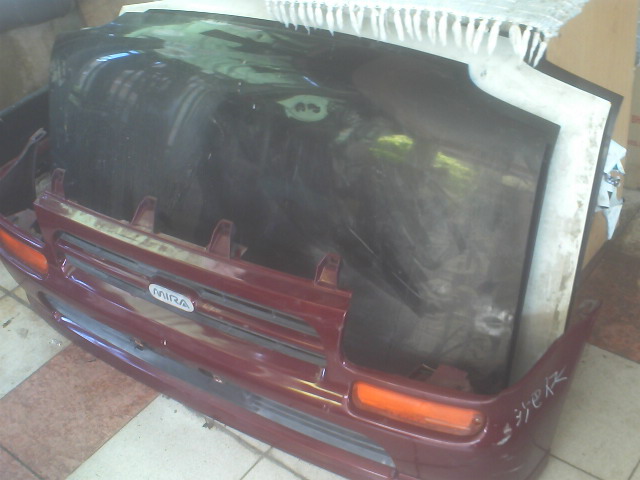This horizontal-rectangular photograph reveals a chaotic scene centered around a car-themed storage organizer, styled as the rear end of a maroon-colored vehicle, adorned with long rectangular orange lights on either side. Prominently featured on the faux bumper is the car manufacturer’s logo, MIRA, spelled out in white letters. The organizer rests on an eclectic tiled floor composed mostly of large white squares interspersed with some medium pinkish-brown and red porcelain tiles. Handwritten white chalk marks trace the side of the bumper. 

Leaning against a beige wall in the background are three car hoods, two black and one white, seemingly placed there for storage or display. Draped above these hoods is a light green blanket with white fringe, slightly casting a reflection on the glossy surface of one of the hoods. Despite a lower quality and some blurriness, the photograph captures the scene effectively, offering a glimpse into this cluttered yet visually engaging arrangement.